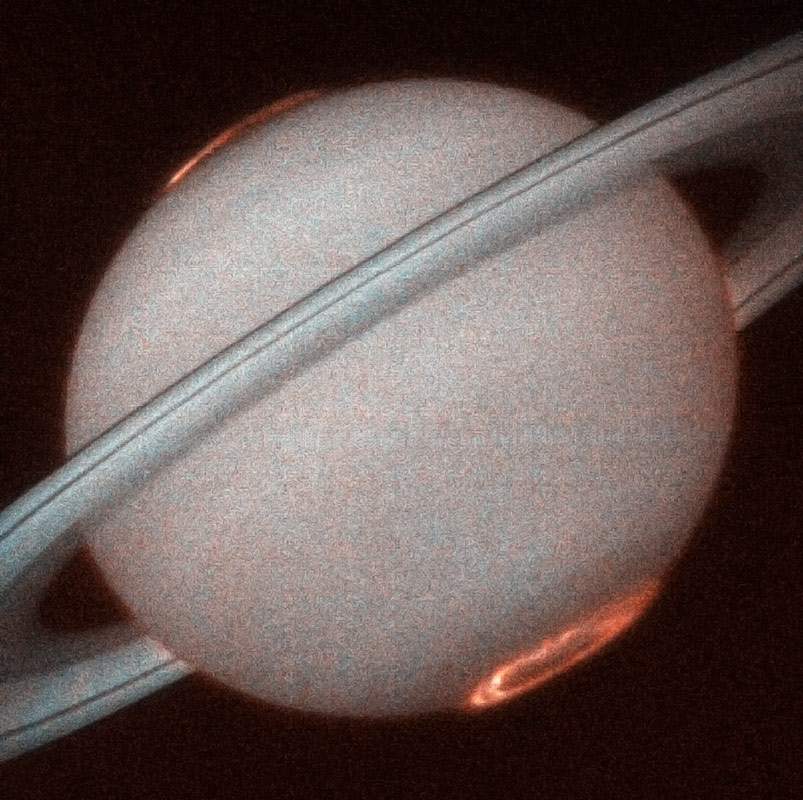This image appears to be a grainy, low-resolution satellite or telescope photograph of Saturn, set against a stark black background with no visible stars. The planet, centrally positioned in the image, initially appears as a large white circle, though closer inspection reveals a mix of subtle light blue and pink hues within the white. The characteristic rings of Saturn encircle the planet, rendered in white with thin gray lines dividing them. The rings cut off at the top left and right edges of the image, tilting slightly to the left. Both the north and south poles exhibit a distinct orange-red glow, possibly indicative of solar storms. This faint, glowing hue creates a subtle halo around the planet, adding to the overall hazy and grainy quality of the photograph.